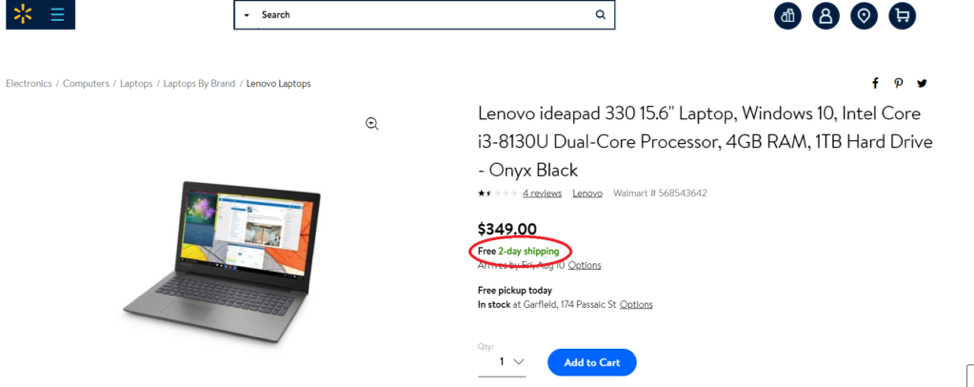This screenshot is from the Walmart website. At the top left corner, there is a rectangular icon - dark blue or black - featuring the signature Walmart yellow spark symbol, centered within a circle. Adjacent to this icon, there are three greenish-blue lines. Towards the center of the header, there is a search bar outlined in black, displaying the word "Search" in black text against a white background. 

Below this header, in tiny grayish text, the navigational path reads: Electronics > Computers > Laptops > Laptops by Brand > Lenovo Laptops. 

A central image showcases a Lenovo laptop, characterized by its very dark gray exterior and black keyboard. The laptop screen displays an image of a flower in a white vase on a table. 

Next to the laptop image, product details are listed as follows: 
- "Lenovo IdeaPad 330, 15.6 inches laptop, Windows 10, Intel Core i3-8130U Dual Core Processor, 4GB RAM, 1TB hard drive, Onyx Black." 
- Customer reviews rating: 1.5 stars.
- Below the reviews, in tiny gray letters, the product identifier "Walmart #5685-43642" is displayed.

The price is prominently shown as $349 with the offer of free two-day shipping, highlighted within a red circle.